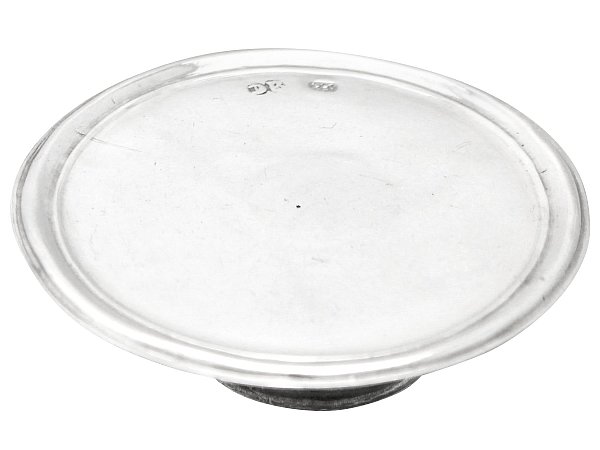This is a minimalist product photograph of a round metal platter, captured in a white void to emphasize the product. The platter, composed of a matte metal, showcases a full view of its smooth, circular surface and part of its base due to the angled shot. The matte finish is accentuated by slight reflections along its edges. Displayed on an understated, low black pedestal, the platter's base appears smaller and rounded, contrasting subtly with the larger upper surface. A maker's stamp, though not clearly recognizable as any specific letter or symbol, is imprinted on the flat end of the platter. The entire composition, isolated against the stark white background, directs the viewer's attention solely to the sleek, understated elegance of the metal platter.